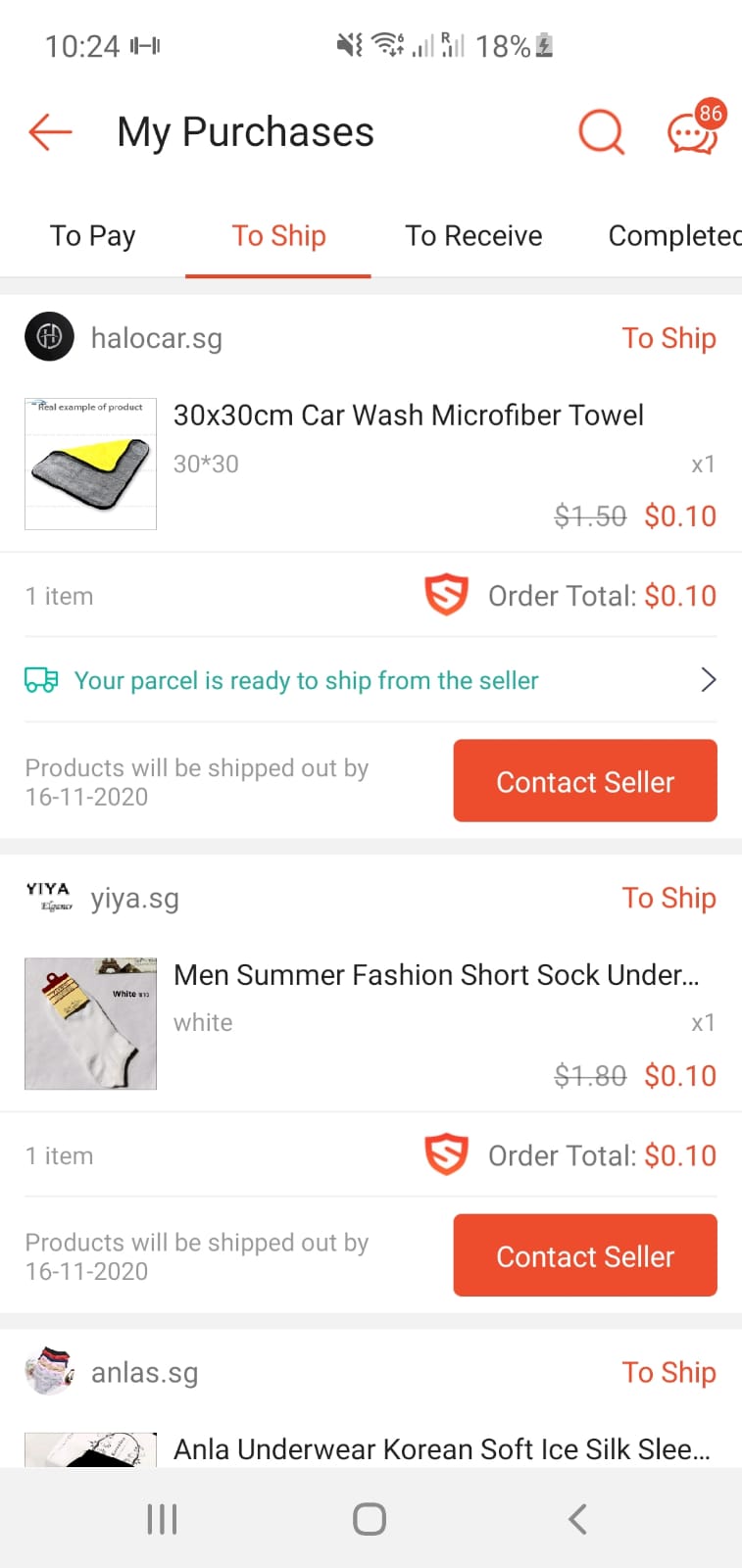A user is browsing their purchases on a shopping app, with the screen displaying the "My Purchases" section. The interface is divided into four tabs at the top: "To Pay," "To Ship," "To Receive," and "Completed." The user is currently on the "To Ship" tab. Three items are visible, although the third item is partially cut off.

1. The first item is a "30x30 cm Car Wash Microfiber Towel," priced at $0.10 after a discount from $1.50. A message states that the parcel is ready to ship from the seller, with an expected shipping date by November 16, 2020. Next to the item description, there is an orange "Contact Seller" button, and the merchant's URL is provided: halocar.sg.

2. The second item is a pair of "Men's Summer Fashion Short Socks," shown as a white sock. Purchased from the merchant yiyay.sg, it is priced at $0.10 after a discount. Only one pair is included.

3. The third item, partially cut off on the page, appears to be another pair of socks from the merchant anlas.sg. Specific details about this item are not fully visible.

Each item includes a brief description, the merchant's name, and the purchase details.